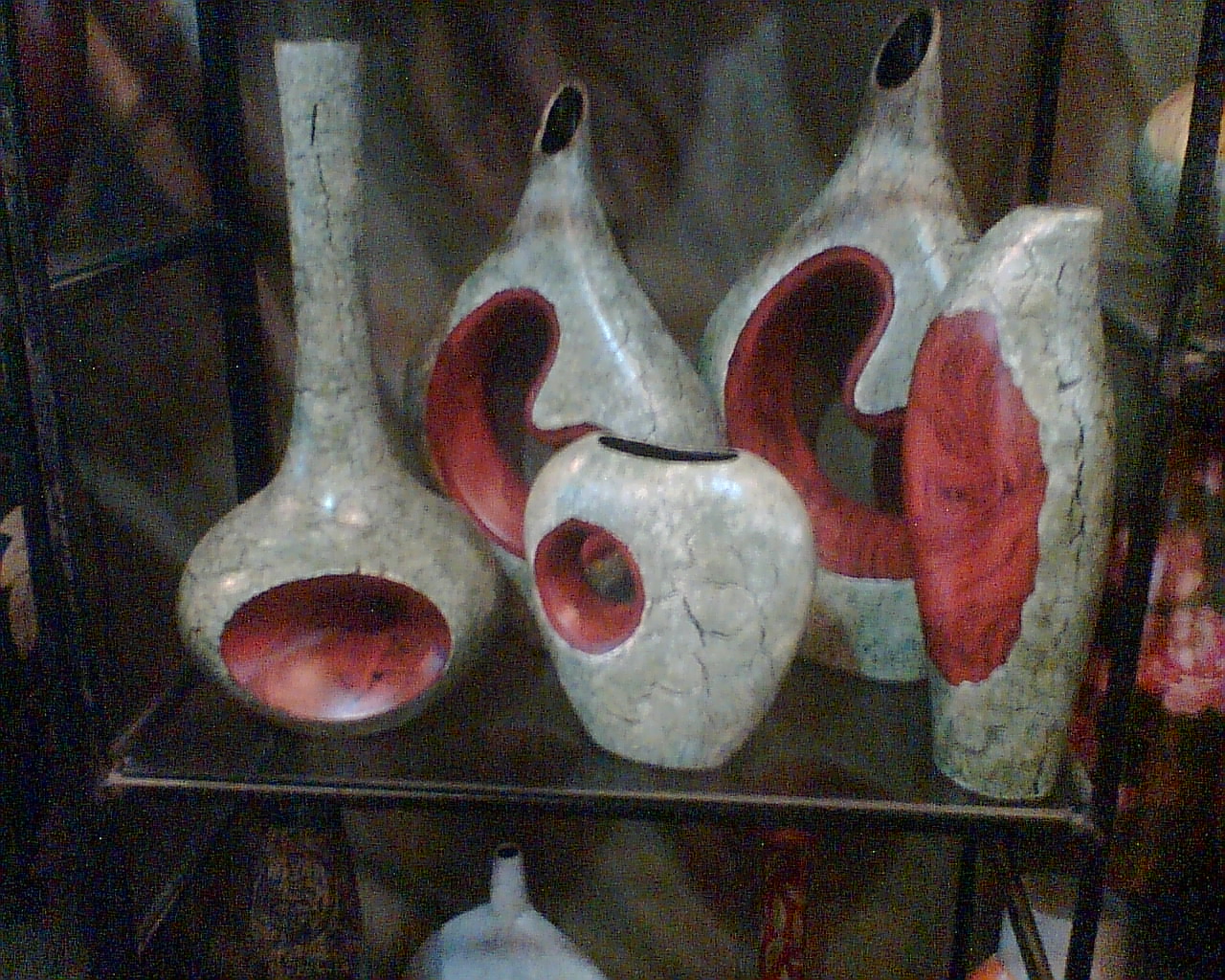This image is a grainy, dark photograph, potentially taken with an old film camera or rendered digitally. It features a glass shelf with five unique, abstract vases of various shapes and sizes, each showcasing a combination of gray, crackled surfaces and striking red interiors. The vases, which appear to be homemade stone or ceramic works, display an assortment of designs: a large bulbous-shaped vase with a long, narrow top, a gray vase with a red indented bottom, and vases with holes that pass through them, revealing red hollows. One vase mimics a hook with intricate shapes, while another has a more traditional, round form accentuated by red in the middle. These vases are empty, suggesting they could potentially hold plants or other decorations. The shelf itself is a dark brownish-black, possibly metal or thin wood. Additional stoneworks and pots are visible at the edges and below the primary display in what appears to be a glass case, set against a brown backdrop adorned with indistinct figures.